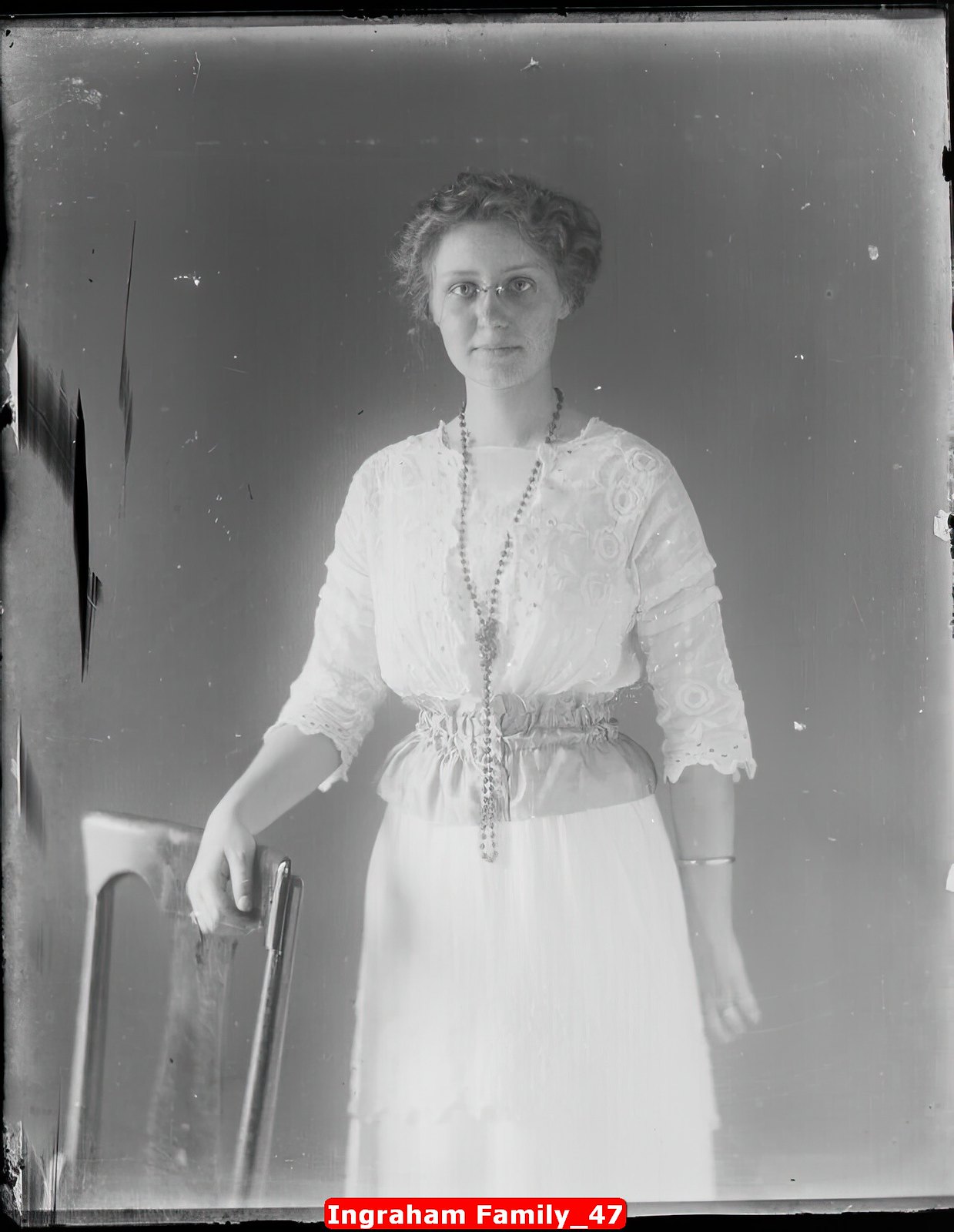This black and white portrait captures a young woman, likely in her 30s, standing and looking directly at the camera. Her dark curly hair is pinned up neatly, and she wears eyeglasses perched on her nose. She is adorned in a white dress, gathered with elastic at the waist, featuring three-quarter-length, lacy sleeves. Around her neck hangs a long, beaded necklace tied in a knot halfway down. The woman's right hand delicately rests on a very old-looking brown chair beside her, while her left arm, decorated with a gold bracelet and a ring, also finds support on the chair's back. The background of the photo is a faded gray, adding to its vintage feel. At the bottom of the image, a label in red with white letters reads "Ingraham Family 47," suggesting it may date back to 1947. The overall appearance of the photograph indicates significant aging and wear over time.